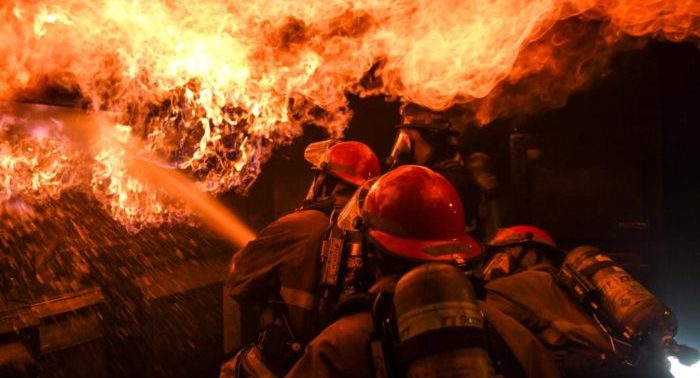This dramatic nighttime photograph captures three firefighters clad in full protective gear, complete with oxygen canisters on their backs and clear visors covering their faces. Their heavy, fire-resistant clothing shields them as they bravely combat a massive blaze that spans the width of what appears to be a building's roof. Positioned with their backs toward the camera, two firefighters support their comrade at the front, who directs a powerful stream of water from a hose towards the intense orange, red, and yellow flames. The inferno, swirling with smoke and dominating the scene, leaves nothing visible beyond the scorching fire and the dedicated firefighters battling to extinguish it.